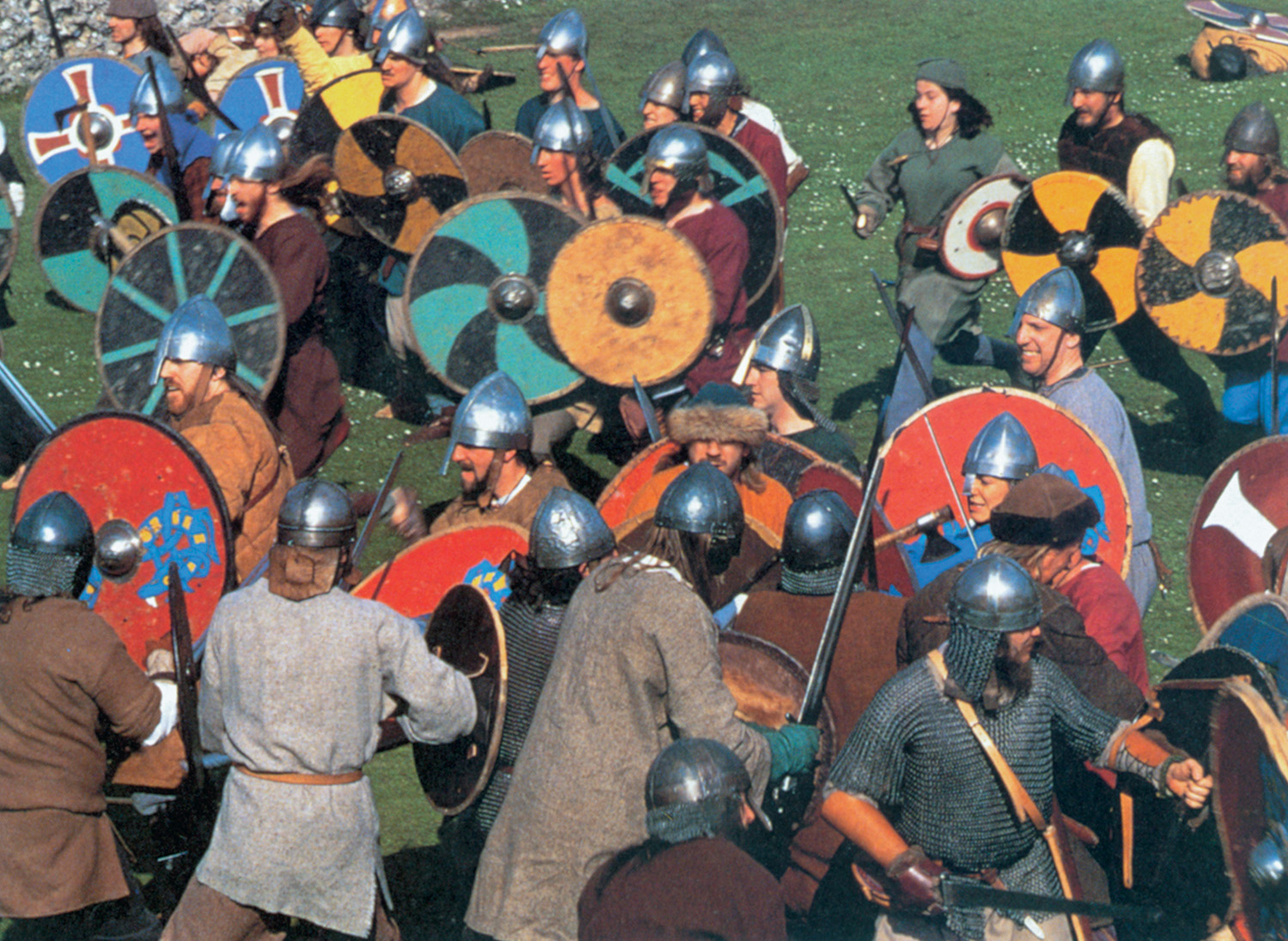The image is a full-color photograph, oriented horizontally, depicting a detailed reenactment of a Viking battle scene. Approximately 20-25 men, predominantly white, are dressed in authentic Viking attire, including chain mail, metal and leather helmets, and capes. They are equipped with swords and spears, showcasing round shields with intricate designs: some shields feature a striking yellow and black pattern, others bear blue with red crosses, while some are solid red or display a teal and black spiral. The battle is staged on a grassy field dotted with small white flowers, possibly clovers. Despite their fierce appearances, several participants are smiling, capturing their enjoyment of the reenactment. In the background, a contingent of about ten men moves leftwards, adding dynamic energy to the scene, while the foreground shows more re-enactors facing towards the background, immersed in the mock combat.